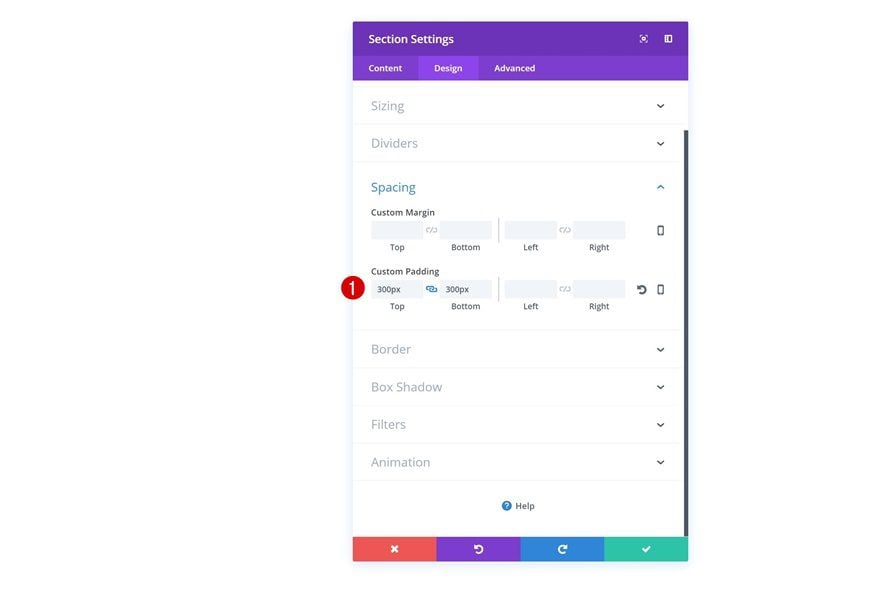Here is a cleaned-up and detailed caption:

A screenshot of the section settings interface displays a user interface with a purple background and white text. The interface features three tabs: "Content," "Design," and "Advanced," with the "Design" tab highlighted. The white screen beneath the highlighted "Design" tab reveals various customization options, including "Sizing," "Dividers," "Spacing," "Border," "Box Shadow," "Filters," and "Animation." 

In the "Spacing" section, there are two primary settings: "Custom Margin" and "Custom Padding." Text boxes for entering values are available for the top, bottom, left, and right margins. In the "Custom Padding" area, a red circle with the number one is displayed, and the values "300px" have been inputted for both the top and bottom padding fields. 

At the bottom of the "Design" tab, a help button is centrally located, followed by a row of four colored action buttons: a red "Close" button, a purple "Backwards" button, a blue "Forwards" button, and a green "Tick" button.